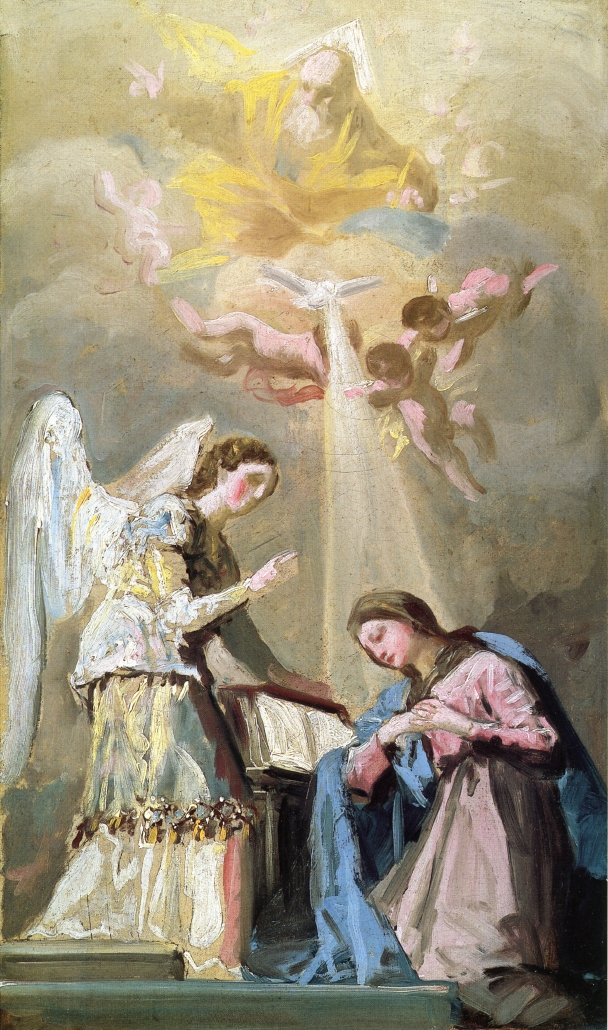The painting captures a serene and divine scene, reminiscent of Renaissance art, with a strong religious undertone. At the center of the sky, a bearded Caucasian man, possibly Joseph or a saint, is depicted wearing a yellow cloak and looking downward. He is surrounded by cherubic baby angels with delicate wings. These celestial beings float among soft clouds and two white doves, which appear to be gracefully flying. Below, on the ground, there is a poignant tableau of two women. The first woman, with angel wings and wearing a flowing gown, stands upright. Beside her, a second woman, dressed in a pink dress and blue robe, kneels with her head bowed in sorrow or prayer. The kneeling woman's posture and attire bear a striking resemblance to traditional depictions of the Virgin Mary. The dove, positioned overhead, softly illuminates the scene below, enhancing the painting's spiritual ambiance. The entire composition, with its gentle hues of blue, yellow, and tan, evokes the grandeur and reverence of classic religious art.